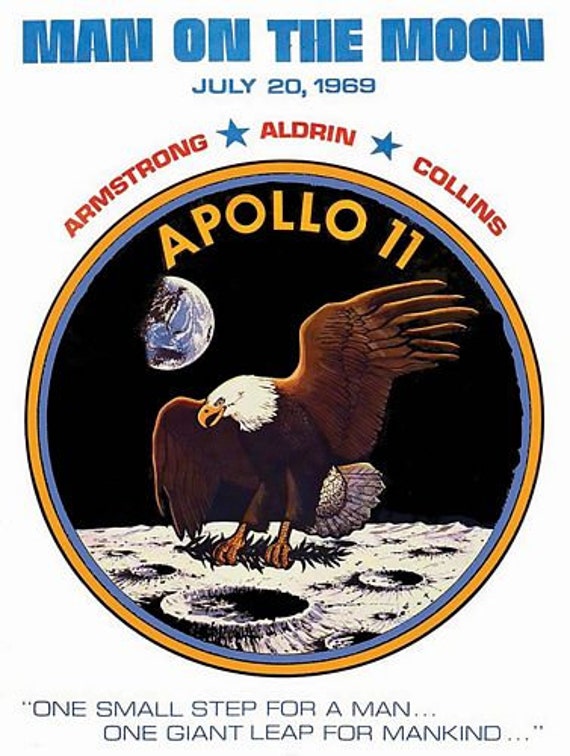A commemorative event poster from the Apollo 11 mission, celebrating mankind's first successful moon landing on July 20, 1969. Featured prominently at the top is the phrase "Man on the Moon," with the date "July 20, 1969" marked in red. Below this, the names of the astronauts – Neil Armstrong (in red), Buzz Aldrin (blue star), and Michael Collins (blue star) – are listed.

The central artwork is surrounded by two circles, one yellow and one blue, adding a decorative frame. The artwork itself depicts the Earth in the background on the left-hand side, providing a striking contrast. At the forefront stands a bald eagle, symbolically carrying items representative of American achievement. The eagle is positioned on the moon's surface. Beneath this powerful image is Neil Armstrong's iconic quote: "One small step for man, one giant leap for mankind."

The poster is likely a celebratory piece created to commemorate the historic mission of Apollo 11 and mankind's incredible achievement of landing on the moon for the first time.